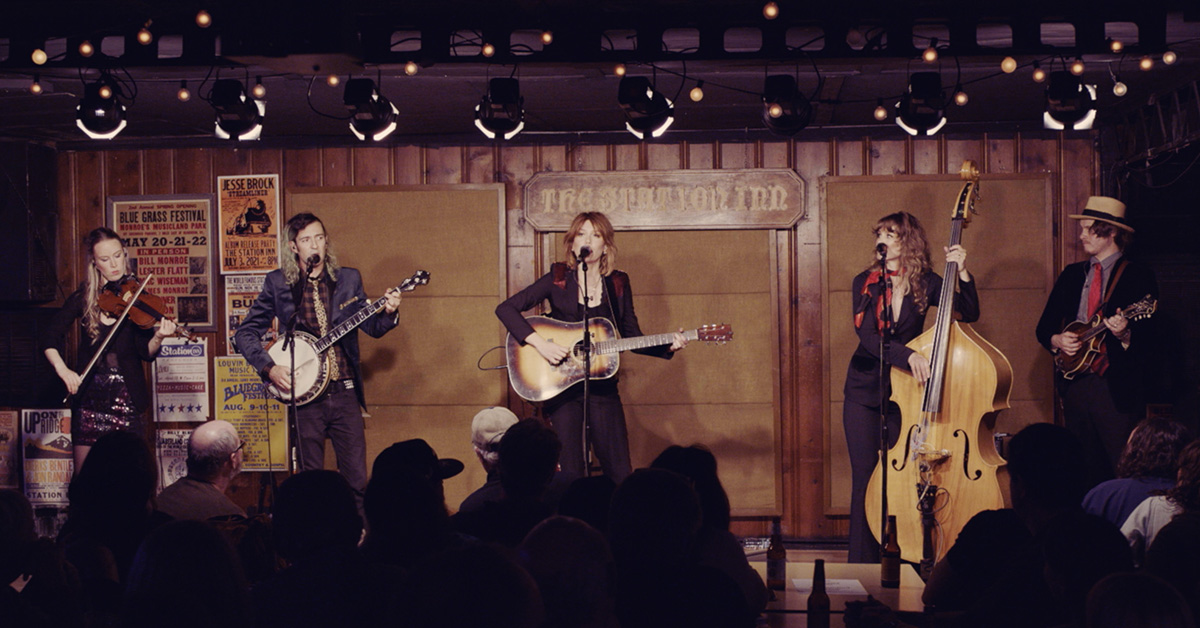In this photo, captured from the back of a silhouetted audience seated around tables, we see a five-member band performing live on stage at "The Station Inn." The band members are dressed in a vibrant, eclectic, and folksy manner, each showcasing unique styles. 

On the far left, a woman with long, blonde hair plays a brown violin, donning a black dress with a sparkly pink skirt. Next to her stands a man wearing a brown suit jacket and blue pants, playing a banjo and singing into a black microphone.

At the center of the stage is a red-haired woman, with blonde highlights, dressed in an all-black female suit, strumming an acoustic guitar. To her right, another woman with curly brown hair, dressed in an all-black suit and a red scarf around her neck, masterfully handles a large bass.

On the far right, a man wearing a black suit with a red tie and a blue-gray collared shirt plays a brown mandolin. The stage is adorned with posters, including one for a bluegrass festival, and is illuminated under spotlights from above, creating a visually dynamic scene. One notable detail in the foreground is a table with three beer bottles, contributing to the lively saloon-like atmosphere of the venue.